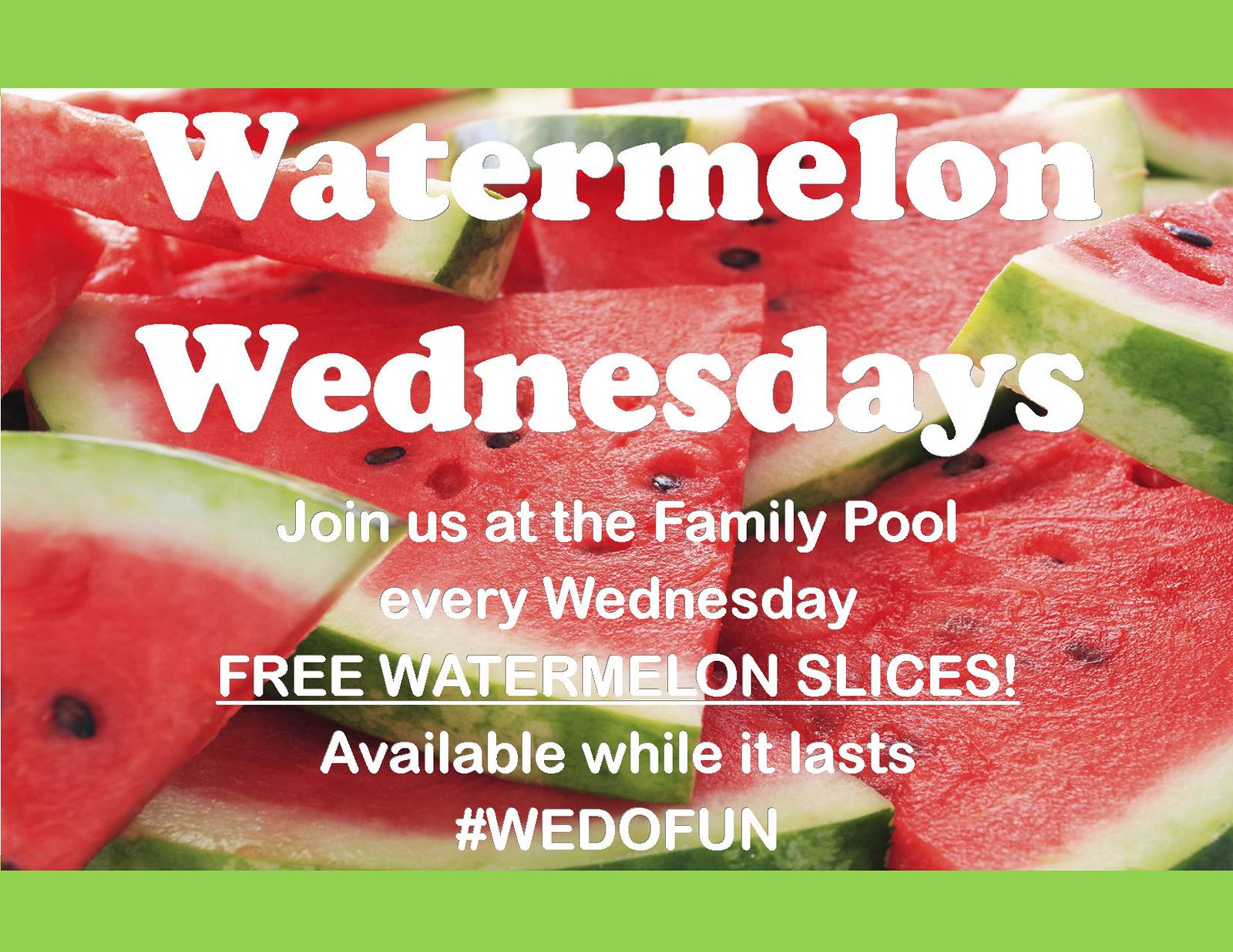The image is a vibrant digital advertisement with a light green border at the top and bottom. The central background showcases a vivid array of triangular watermelon slices, giving the image a fresh and appealing look. Prominently displayed in large white font are the words "Watermelon Wednesdays". Beneath this, it invites viewers to "Join us at the family pool every Wednesday" in slightly smaller white text. Emphasized in all caps, underlined, and with an exclamation point, the ad promises "FREE WATERMELON SLICES". Below, it notes "available while it lasts". Concluding the message in all caps, it reads "HASHTAG WE DO FUN". This appealing and well-designed advertisement aims to attract families to the pool on Wednesdays for free watermelon.